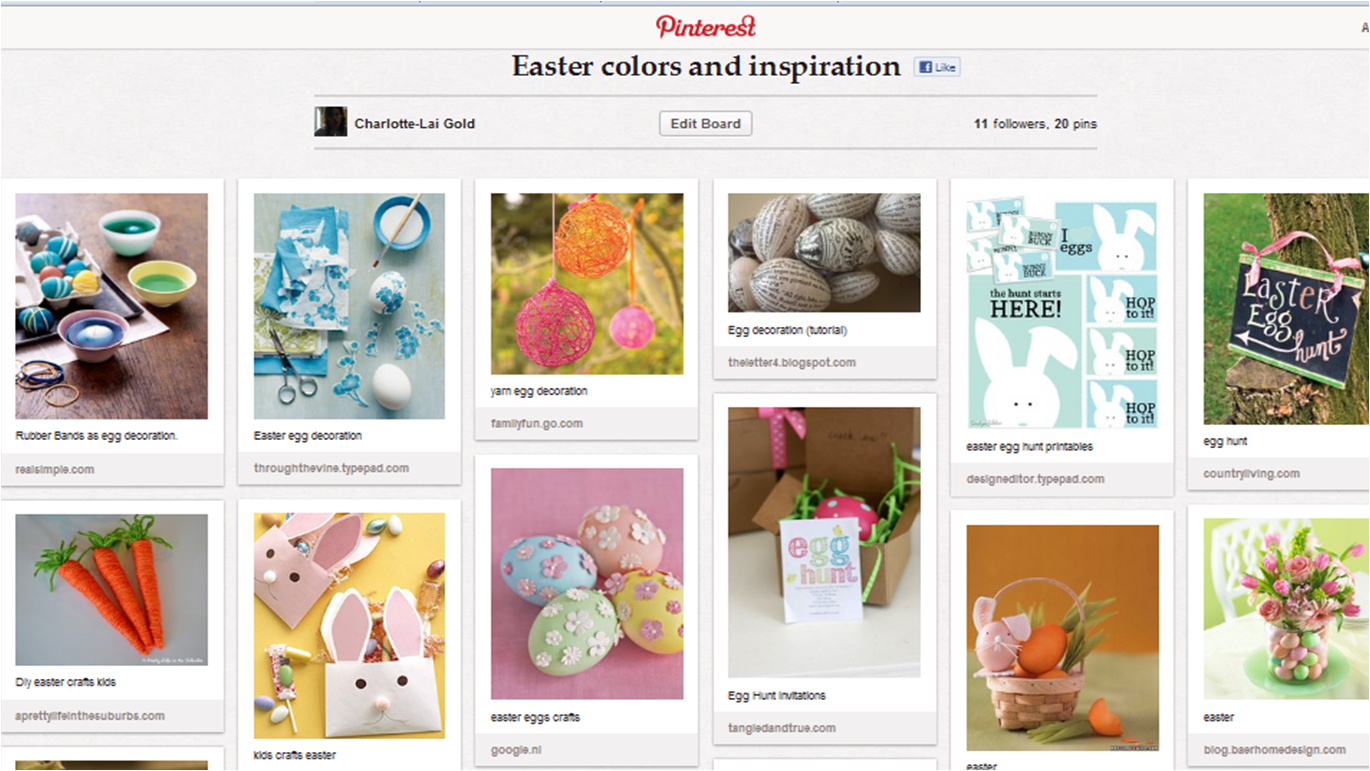This is a detailed screenshot of a Pinterest page with a light gray background. At the top, there is a white bar featuring the word "Pinterest" in red font. Below this, a black line is followed by text in black font that reads "Easter colors and inspirations." To the right of this text, there is a 'Like' button. Another black line below this section states "Charlotte Lie Gold, Edit Board, 11 followers, 20 pins."

Displayed beneath this information are two rows of Pinterest pins, each consisting of small labeled pictures. Each image comes with a brief description and indicates its source. All the pictures are Easter-themed.

In the upper left, there's an image of a brown table with bowls of egg dye and eggs being dyed. To its right, another image shows a white table where eggs are having paper glued to them. Continuing to the right, there are pictures of hanging egg ornaments. Further right, there is an image of eggs decorated with words written on them. The final image on the far right features little bunnies.